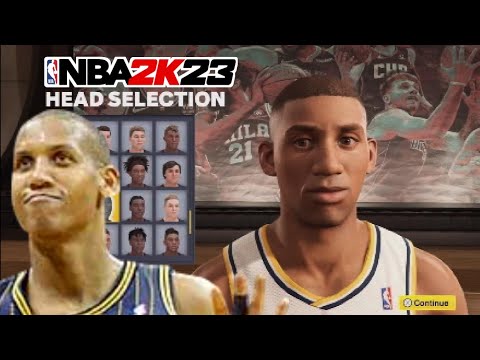A detailed in-game screenshot from an NBA video game, presented in a widescreen format with thin black bars framing the top, bottom, left, and right edges. Prominently displayed in the background are NBA players, including a team on the right side wearing black jerseys with white text. These players, all African-American, are poised with orange basketballs, ready to shoot. To the left, the iconic NBA logo, featuring a white silhouette of a player with a ball against a red, white, and blue background, is prominently displayed. Adjacent to the logo, white and black text spells "NBA," followed by "2K" in bold red, and "23" in black, with the phrase "head selection" in smaller white text beneath.

In the lower left section of the image, a bald African-American player in a purple and yellow jersey looks upwards with a confident demeanor. To the right, possibly a different character, though intended to be the same, has a full head of hair and a distinctly different facial structure, donned in a jersey with a white base and purple and gold trim. At the bottom right corner, a yellow rectangle featuring a white 'X' and the word "continue" in black text invites the player to proceed. The notable differences in the depicted characters, despite indications they might be the same, suggest a visual disparity often encountered in video game representations.